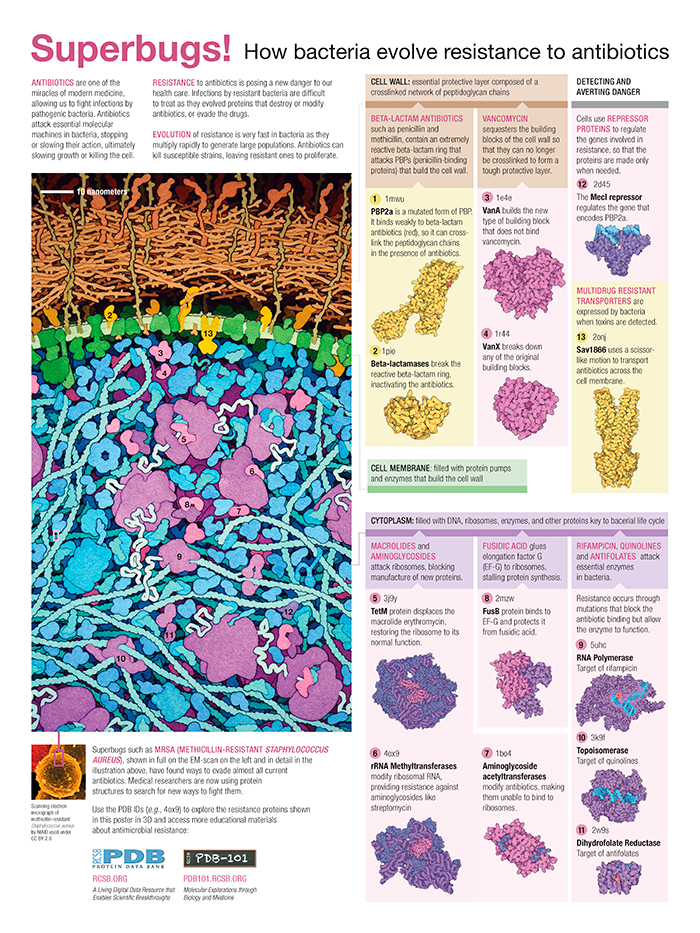This image showcases an informational science poster titled "Superbox: How Bacteria Evolve Resistance to Antibiotics." The poster is densely packed with various digital artworks and text detailing the mechanisms behind bacterial resistance to antibiotics. 

At the top, prominently highlighted in pink, is the word "Superbox," followed by the subtitle in black text, "How bacteria evolve resistance to antibiotics." Although some of the smaller texts in black and purple are illegible, they likely contain additional details supporting the main topic.

The left side of the poster features intricate digital illustrations of bacteria at a microscopic level. These images include a large, rounded cell wall filled with blue and purple masses, representing different cellular structures and components. Above this are layers of intertwining brown strands and a green layer, illustrating various molecular interactions within the cell.

On the right side of the poster, there are colorful masses—some deep purple, light purple, and yellow—depicting bacterial proteins and molecules. These vibrant illustrations aim to visualize the complex processes of bacterial resistance mechanisms. Overall, the poster combines detailed imagery and informative text to educate viewers about how bacteria develop resistance to antibiotics over time.